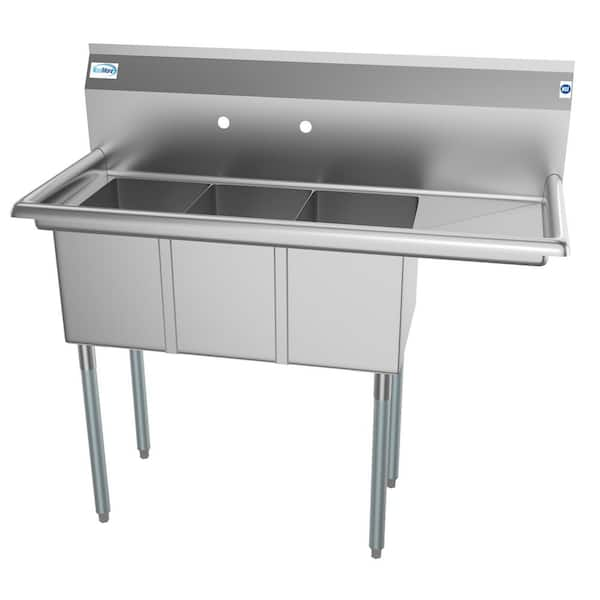This is a professionally staged product photo of a commercial-grade industrial sink typically used in large kitchens, such as those found in restaurants or hotels. The sink is made of polished silver metal, possibly stainless steel or aluminum, and features four sturdy legs that support the unit. The main section includes three deep, rectangular basins suitable for washing various items, similar to the setup found in restaurant prep areas like Subway. To the right of the basins is a small counter space. The back of the sink has two holes, presumably for pipe installations. The photo is taken against a white background with studio lighting, ensuring no distracting reflections on the polished surface. There are small, unreadable stickers or logos on the left and right sides of the sink.